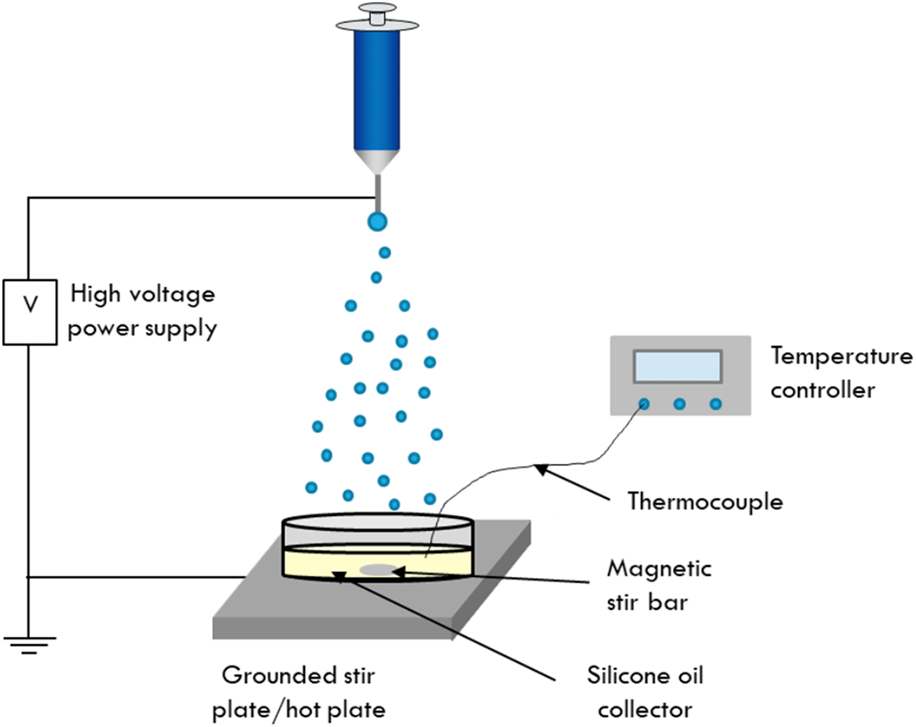This horizontal diagram illustrates the functioning of a scientific apparatus. At the top, a syringe filled with blue liquid is depicted, dispensing blue droplets one at a time. Connected to the syringe is a label reading "High Voltage Power Supply," which is grounded for safety. The blue droplets fall into a circular container filled with a yellow liquid, labeled "Grounded Stir Plate / Hot Plate." The container is equipped with a magnetic stir bar for mixing the liquid. 

On the right side of the container, a temperature controller is shown as a gray rectangular box, with a display and three blue dots. A thermocouple connects the temperature controller to the yellow liquid to measure its temperature. The label "Thermocouple" indicates this connection. Below this, black arrows point to various components, highlighting their functions. Lastly, underneath the apparatus, a "Silicone Oil Collector" is indicated, showing where excess silicone oil is collected during the process. The entire diagram consists of black and blue lines, providing a clear and detailed representation of the equipment and its components.